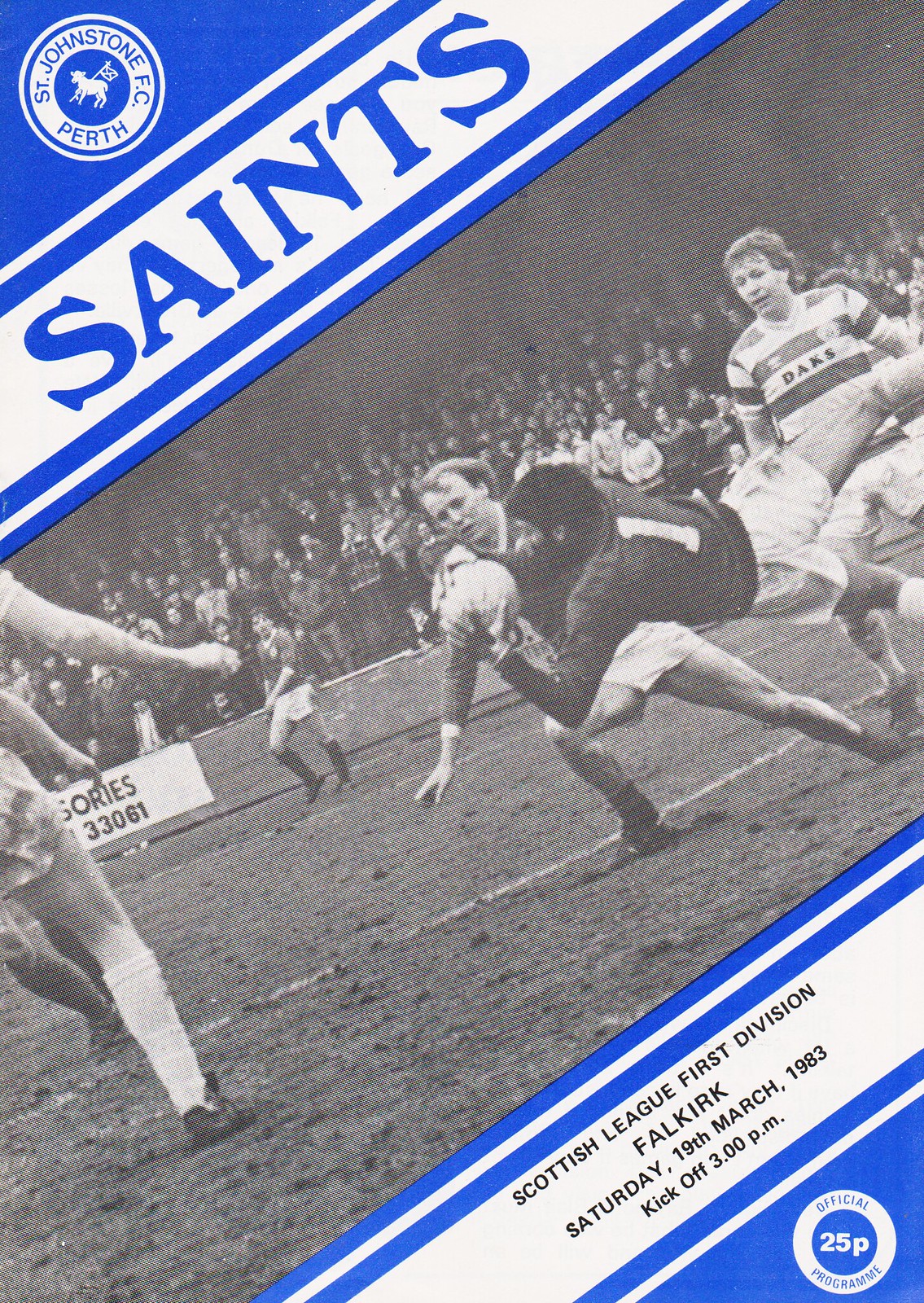The image is the cover of a vintage St. Johnstone F.C. Perth program from a soccer match. The design features a black-and-white photograph of an intense game with a goaltender diving to catch the ball, surrounded by other players. The background reveals stands filled with spectators. Identifying details are located diagonally across the cover. At the top left, there's a blue triangular section featuring the club's logo, a white circle with an animal and a flag, encircled by the text "St. Johnstone F.C. Perth." Below this, a white banner with bold blue lettering reads "Saints." Meanwhile, the bottom right contains another blue diagonal section with a white banner indicating "Scottish League First Division Falkirk, Saturday 19th March 1983, kickoff 3 p.m." Additionally, within the bottom right corner, a white circle displays "Official Program 25P" in blue text. The overall style is reminiscent of 1980s print media, strikingly simple yet informative.